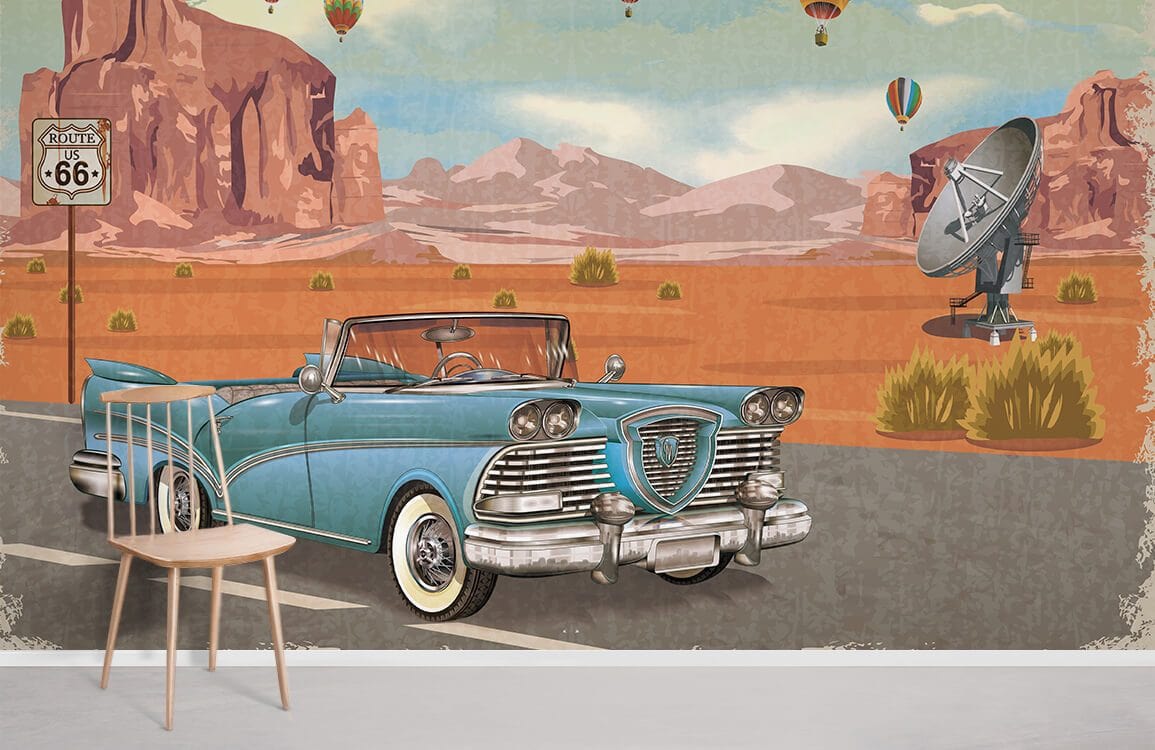The image depicts an indoor scene dominated by a large, horizontally aligned rectangular picture, possibly a painted wall or a large poster. In the foreground on the left side, there's a small light brown wooden chair positioned on a light gray floor, which fades into a white baseboard at the bottom of the image. The wall behind the chair features a detailed depiction of a desert landscape.

At the center, an old-school turquoise convertible, reminiscent of a 1950s style car, is parked on a gray road marked by white dashed lines. The car has white-walled tires, a silver bumper, and dual headlights; there is no passenger inside.

To the left of the car, a Route 66 sign is prominently displayed, while a large gray satellite dish stands to the right. The desert terrain is dotted with spiky green plants, possibly cacti. In the background, several mountains and cliffs create a layered horizon, transitioning from shades of brown and pink to faded silhouettes in the distance. The sky is partly cloudy with white and gray clouds interspersed with patches of blue. Adding a whimsical touch, several hot air balloons float above the mountainous backdrop, enriching the overall scenic and nostalgic ambiance of the image.